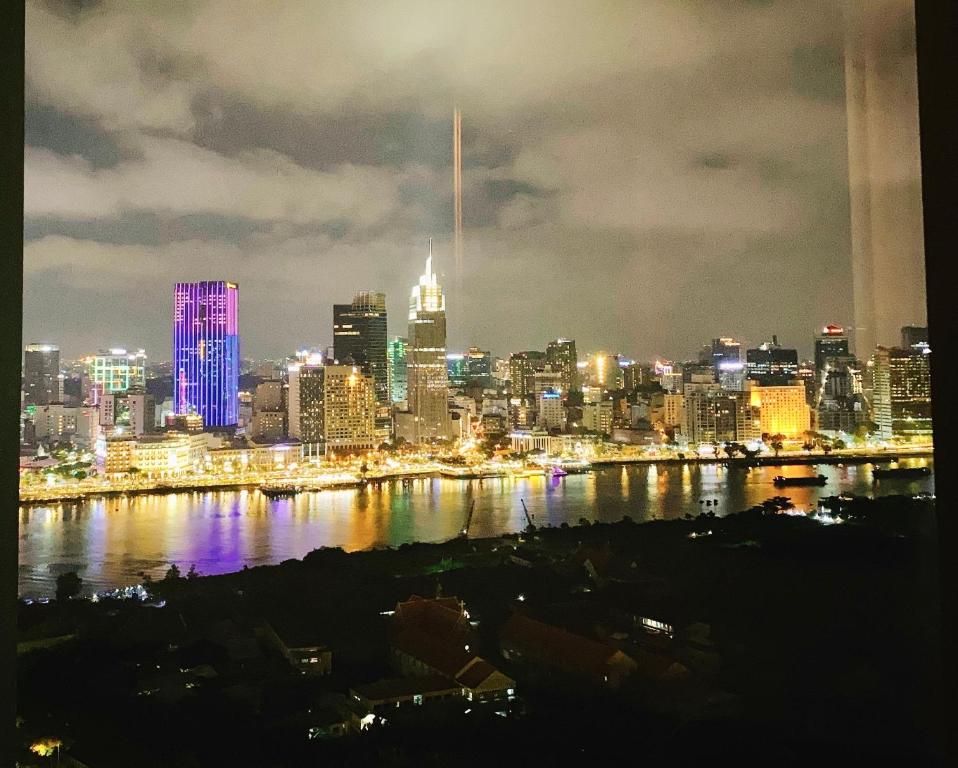This detailed nighttime photograph captures a vibrant cityscape illuminated under what appears to be a very bright moonlight. The view, taken from a high vantage point, reveals a contrast between a dark, low-lying residential area in the foreground and a brightly lit city skyline in the background. The immediate foreground is populated with dimly lit structures, including a few notable buildings with red roofs and some trees, although much of this area is shrouded in darkness.

At the edge of this residential area, there are cranes and two barges visible on the right side of the river, which runs horizontally through the photograph. The black silhouettes of the barges and the dark riverbed add depth to the scene. The river itself acts as a mirror, reflecting the myriad lights from the skyscrapers across the water, which sparkle in hues of purple, yellow, green, orange, and more. 

The cityscape along the far bank is densely packed with skyscrapers of varying heights, many of which are intricately illuminated. Notably, one tall rectangular building is lit with electric blue at the bottom and purple at the top, with its vibrant reflection mirrored in the river below. Another prominent skyscraper in the center of the image features a top that glows pure white. A brightly lit roadway along the riverbank further accentuates the city’s luminosity.

The sky above is cloudy, adding a dramatic backdrop to the scene, with beams of orange light from city spotlights piercing through the clouds. On the right side of the photograph, some additional distant lights create a soft, blurred effect, contributing to the overall sense of depth and perspective in this breathtaking night scene.